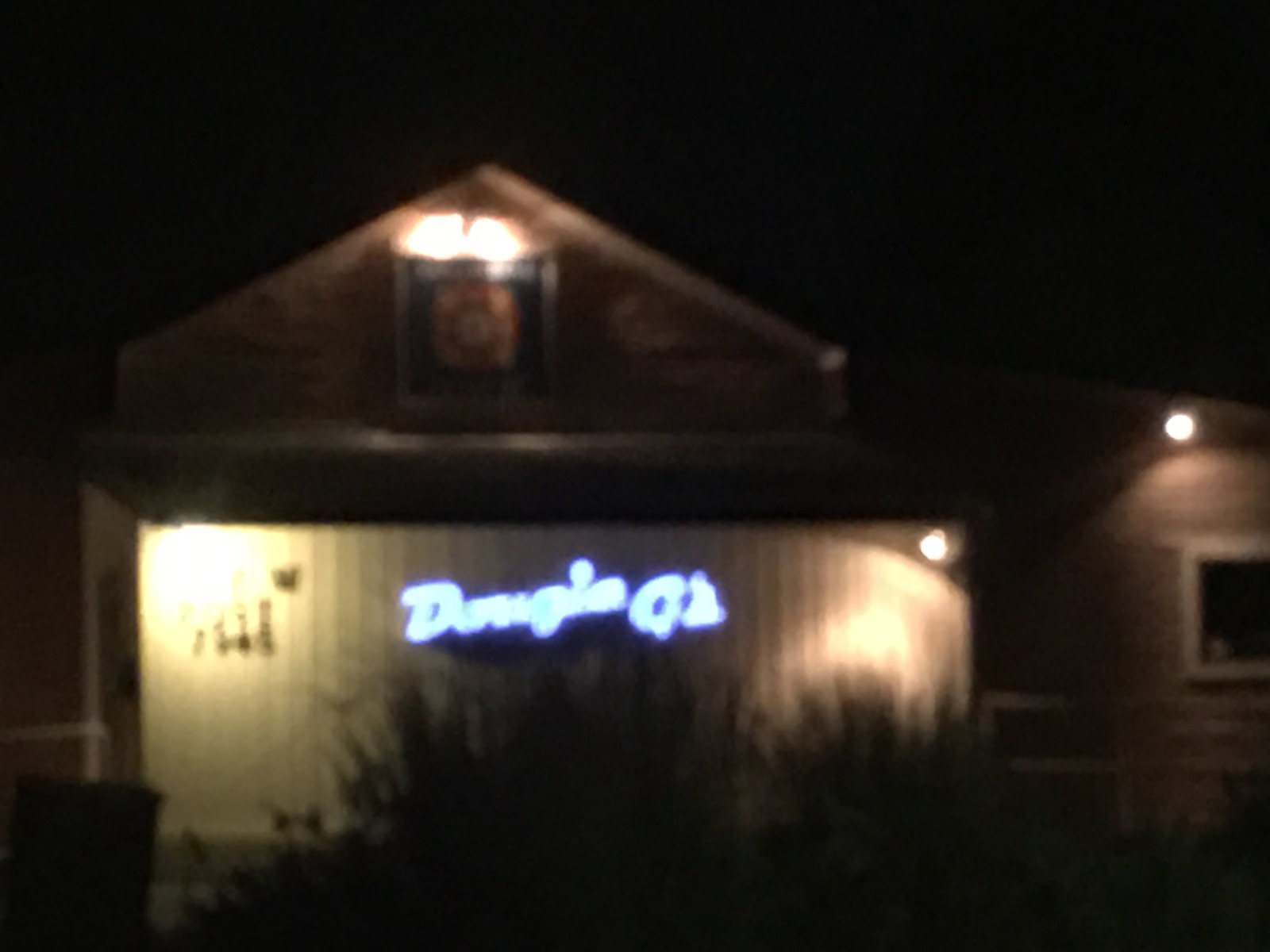In the image, there is a one-story building with an additional half-story above it. The exterior features a white door adorned with black elements, and the entryway is warmly illuminated. Above the door, a neon sign begins with the letter "D," but the rest of the text is indecipherable due to the picture's blurriness. The porch area is well-lit, revealing tall vegetation growing in front of the building. At the peak of the roof, there is a lit sign or flag, but it is also too blurry to clearly identify.